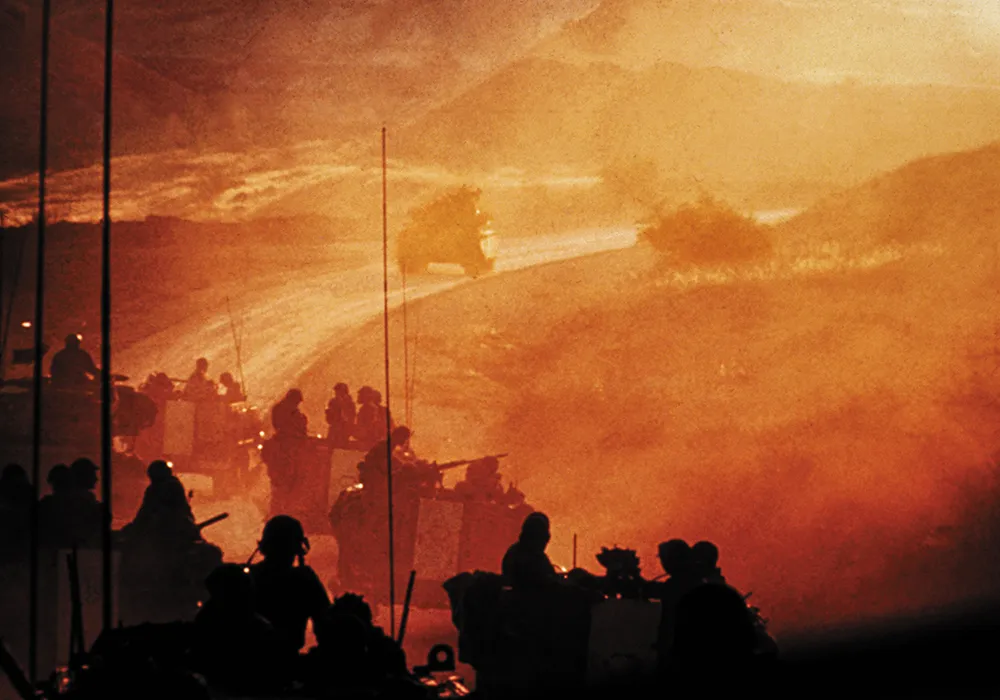The image portrays a convoy of military vehicles traveling on a desert-like road during either dusk or sunrise, evidenced by the hazy lighting and the slight yellow hue over the black-and-white photograph. In the foreground, multiple military vehicles, each manned by around three to five soldiers, are equipped with mounted guns and are spaced along the dusty road that winds towards the horizon. A single tank leads the convoy at the top center of the image, driving past a small hill that slopes gently upwards at approximately a 15-degree angle on the right side. Antennas are visible protruding from the vehicles, reinforcing the military aspect. Despite the blurriness of the photo, possibly indicative of an older image or a negative, details such as the silhouettes of the soldiers, their vehicles, and scattered desert shrubs are discernible. The image captures a moment of movement and readiness against a backdrop of a stark, slightly hilly desert landscape.